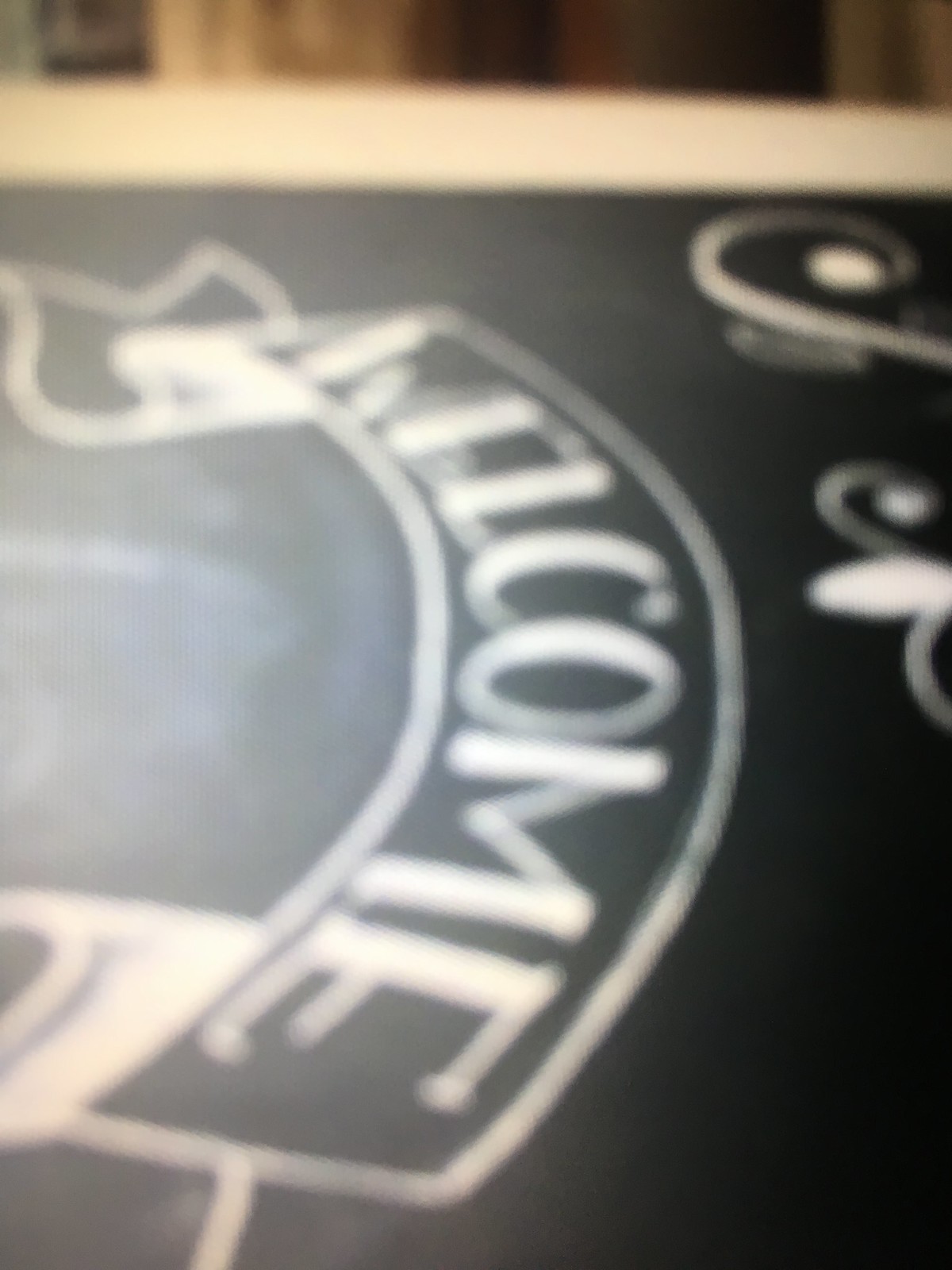The image is a blurry, close-up photograph of a black sign with a white frame that appears to be turned on its side. The sign has a chalkboard-like surface, with a prominent "WELCOME" message in white block letters displayed across a ribbon-shaped banner in its center. Above the banner, there is a geometric flower-like design that is faintly visible. The top portion of the image (which is the right side of the sign) features decorative swirls, each ending in large round areas. Additionally, the background shows a brown and white surface. The photograph has a white shadowing effect beneath the "WELCOME" banner and a white residue that gives it a slightly erased chalk look.